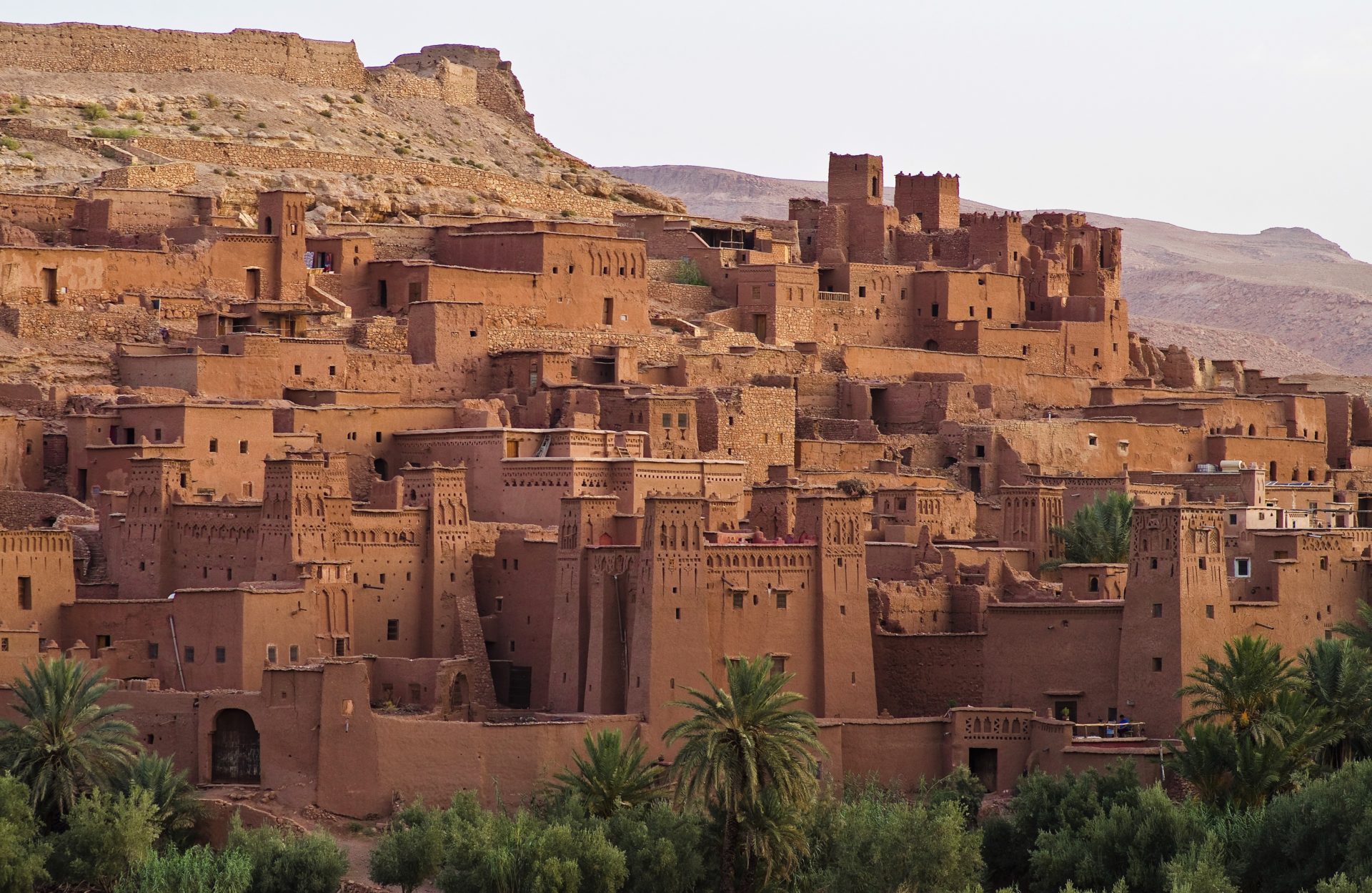This captivating photograph showcases an ancient city built into the side of a hillside, likely located in the Middle East. The city is composed predominantly of brown and red clay or brick buildings that blend seamlessly into the rugged terrain, giving it an earthy, monochromatic palette with shades of light and dark browns. The hillside itself seems to transition into a flat, plateau-like summit.

In the lower portion of the image, a variety of greenery, including palm trees and other tree species in shades of dark and light green, provides a striking contrast against the muted browns of the buildings. Noteworthy architectural features include square windows, multiple archways, and entranceways scattered throughout the city. Particularly prominent is an archway in the lower left corner that appears to serve as an entrance to the city or fortress. Another square archway on the right side suggests additional access points within the city's walls.

The background of the photograph reveals distant mountains, enhancing the sense of depth and location. Several turrets or towers are visible among the buildings, further emphasizing the historic and possibly fortified nature of this site. No visible roads or modern infrastructure can be seen, reinforcing the ancient and preserved character of the city. This image, likely a travel photograph, beautifully captures the essence of an ancient, semi-tropical Middle Eastern hillside city, steeped in history and architectural splendor.